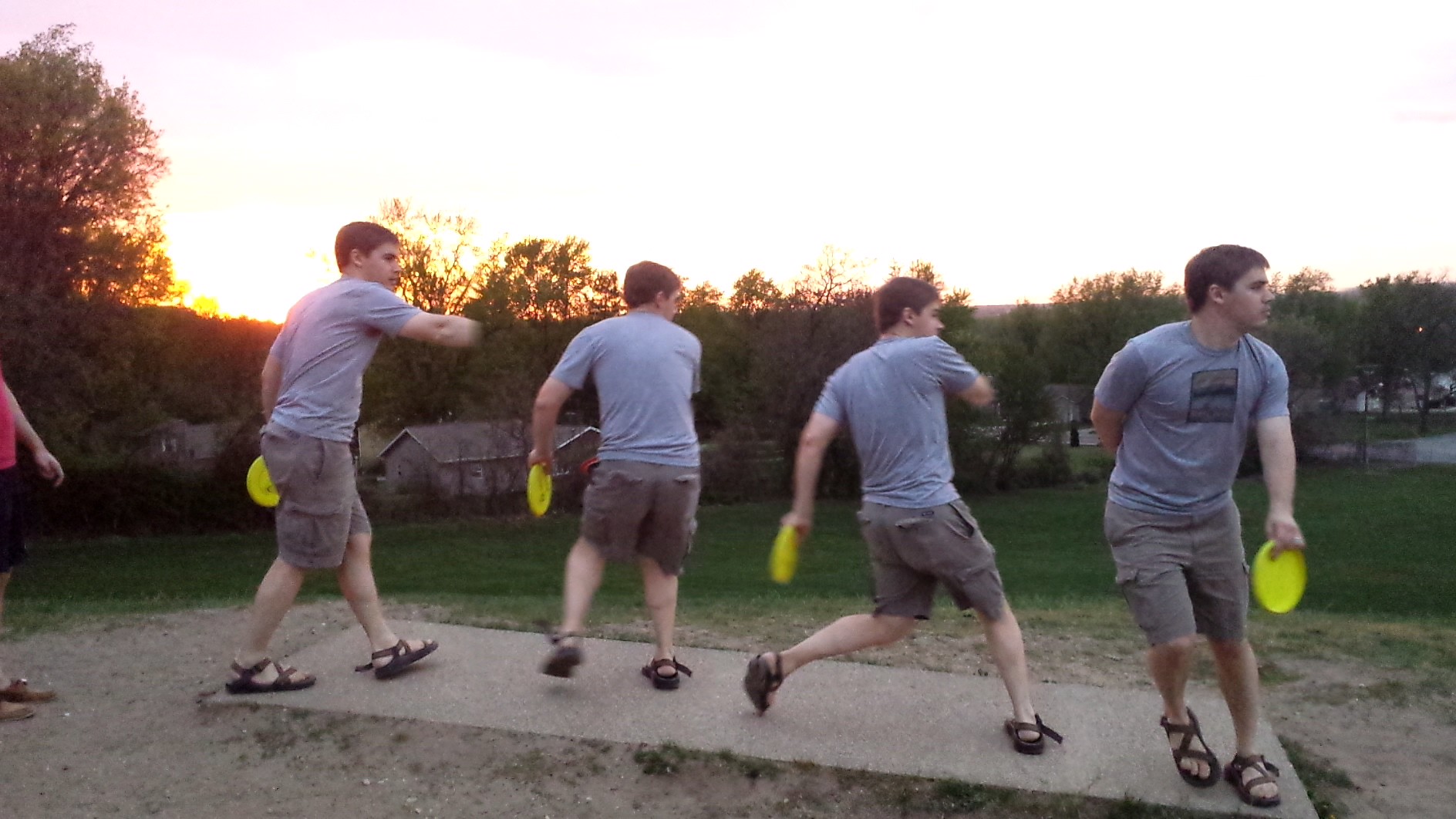This image is a detailed time-lapse sequence showing a young man engaged in the act of throwing a yellow frisbee, possibly during a disc golf game. The sequence captures him in four distinct stages of his throw. The young man is standing on a rectangular cement slab set amidst a sandy area surrounded by patchy grass. In the first stage, he is seen with the yellow frisbee held down by his left side, his right side facing the camera. The second image shows his back to the camera, his legs slightly bent, still clutching the frisbee in his left hand. The third stage captures him from the side, taking a large step forward, preparing for the throw. In the final stage, he appears to have just completed the throw, now facing the camera, though the frisbee remains in his hand, suggesting a practice motion.

The photograph is taken at either sunrise or sunset, with the sun just peeking over the horizon, casting a warm glow over the scene. The young man is dressed in a bluish-gray t-shirt with a graphic on the front, gray cargo shorts with multiple pockets, and brown strappy sandals. His light skin and short brown hair are visible. In the background, there is a field bordered by lush green trees and residential houses. To the left edge of the image, a partial view of another person is visible, showing their shoes and an extended arm, which could indicate onlookers or officials near the scene.